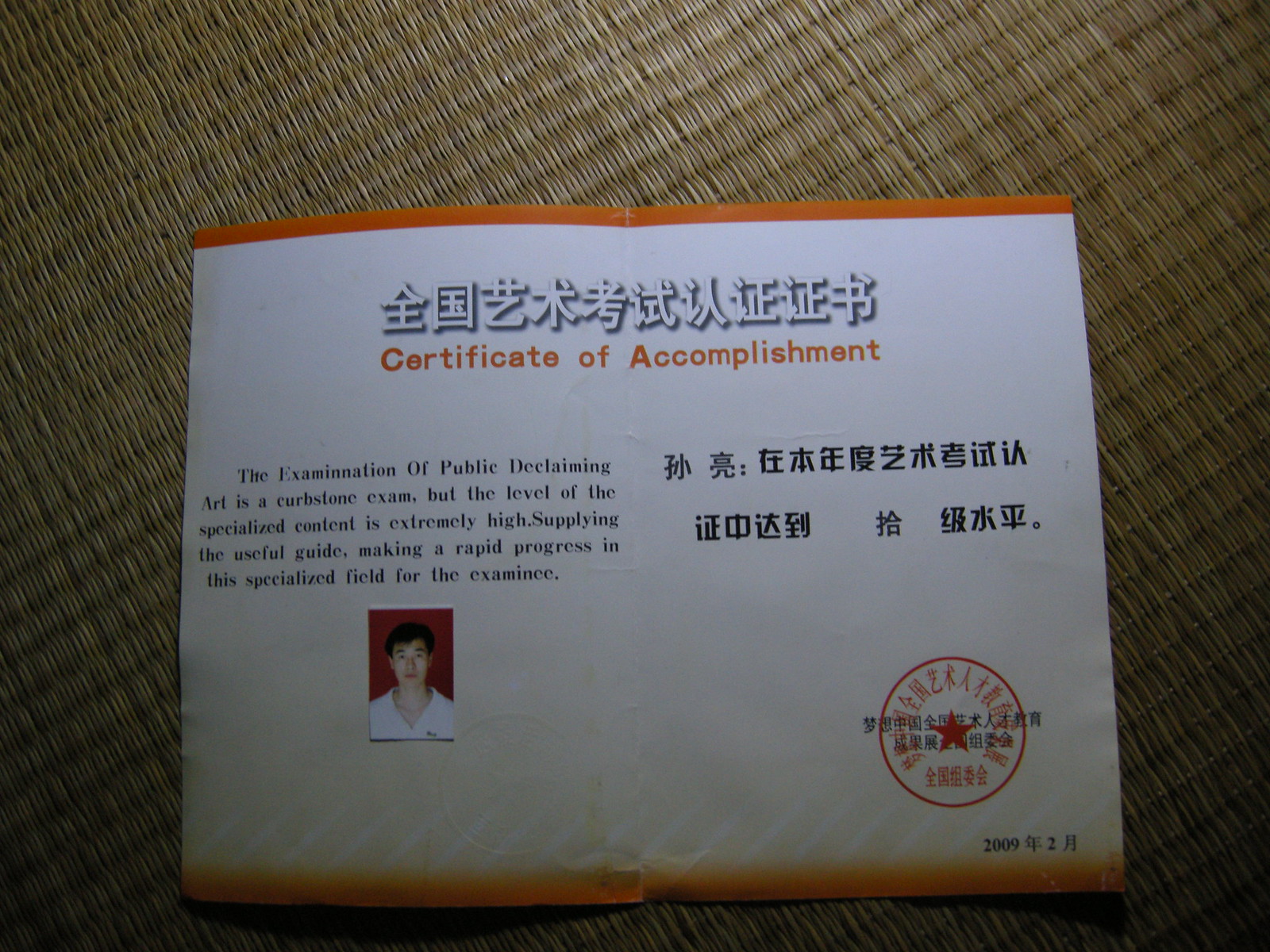The image depicts a Certificate of Accomplishment, prominently placed at the center against a tan rug background. The certificate, roughly the size of a standard sheet of paper, features a predominantly white background with an orange frame adorning the top and bottom edges. At the top, a line of Japanese characters is displayed above the English text "Certificate of Accomplishment" written in orange. Below this, on the left side, a paragraph in English reads: "The examination of public declaiming art is a curbstone exam, but the level of the specialized content is extremely high, supplying the useful guide making a rapid progress in the specialized field for the examinee." On the right side, there are two lines of Japanese text. The lower section includes a small portrait of an Asian man on the bottom left and an official seal featuring a circle and star on the bottom right. The overall setting suggests a moment of recognition, celebrating an individual's achievement in a specialized field.